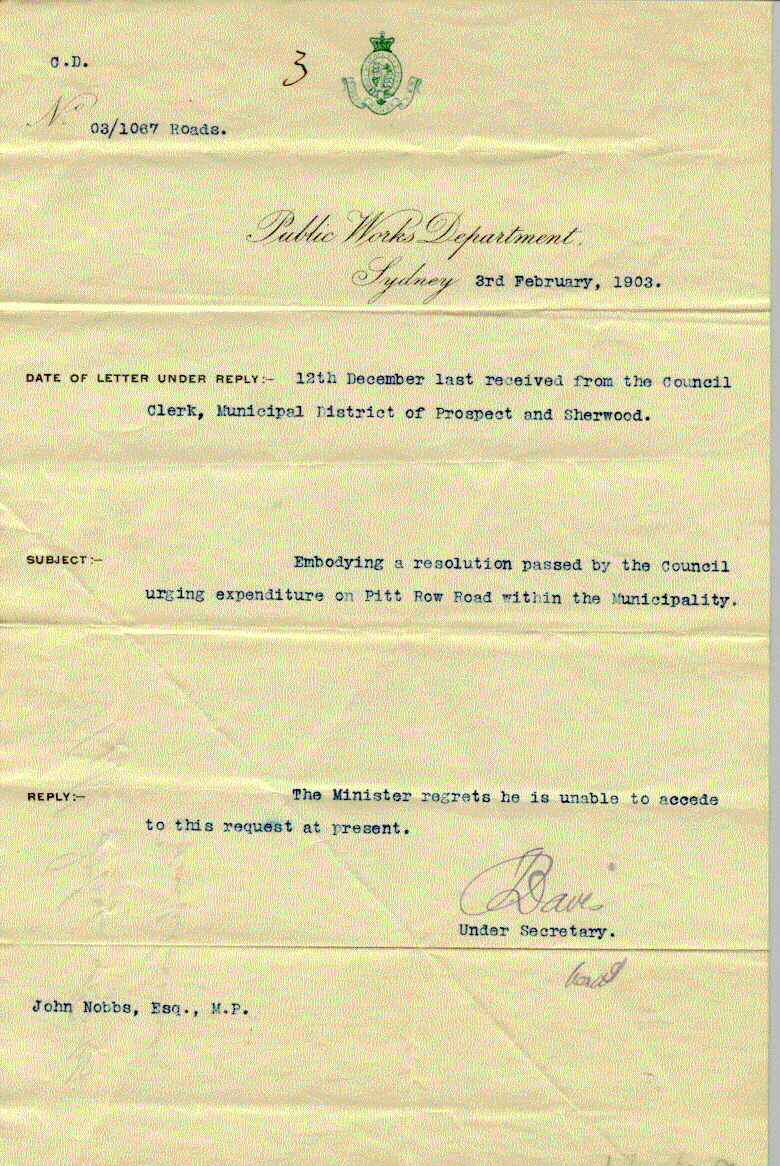The image features an official-looking letter, prominently occupying the entire photo on a parched brown paper background. At the top left corner, there is an indistinguishable abbreviation ("OD" or "CD"), followed by handwritten script "NO." Below this, a line reads "03/1067 Roads." There is a green crest or logo at the top, adjacent to the digit "3." The letter is issued by the "Public Works Department, Sydney," dated "3rd February 1903."

The letter elaborates on its subject matter with a formal structure: "Date of letter under reply: 12th December. Last received from the Council Clerk, Municipal District of Prospect and Sherwood." This is followed by a typed subject: "Embodying a resolution passed by the Council urging expenditure on Pit Row Road within the municipality." The reply reads, "The Minister regrets he is unable to accede to this request at present." Underneath is a signature area, with the typed name and title "Under-Secretary."

In the lower left corner, the letter is addressed to "John Knobs, Esquire, M.P." The text reflects the formal municipal communication style typical of the early 1900s, and the colors in the image include tan, black, grey, green, and brown, adding to the aged appearance of the document.